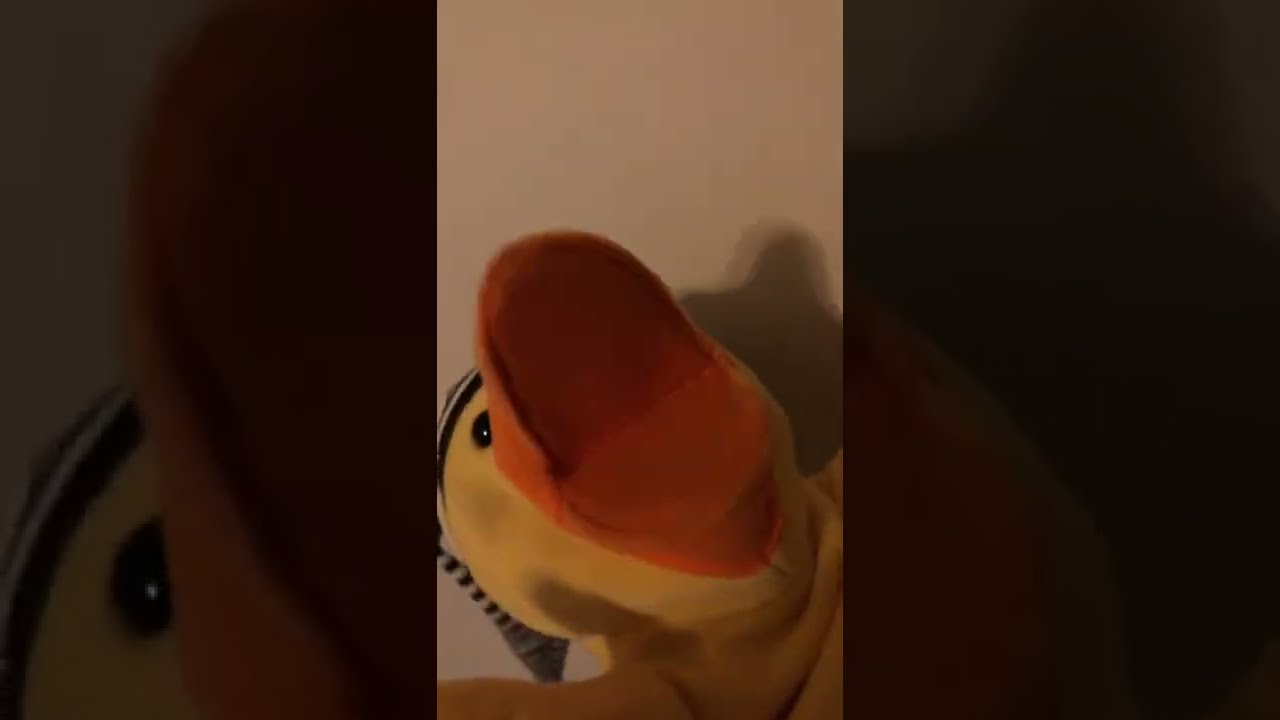In this indoor image, a single stuffed yellow duck is positioned towards the bottom against a solid white backdrop. The duck lies flat on a smooth surface and looks upward with its orange beak wide open, creating a clear view of its mouth. Only one of its black eyes is visible, partially obscured by the beak. The duck sports a hat adorned with black and white stripes. Alongside the duck and the shadow it casts on what appears to be a bridge wall, the setting and colors—off-white, orange, yellow, black, and gray—indicate an environment with ample lighting, likely during the day. The composition includes a split-screen effect, with the central image brightly illuminated and flanked by darker, shadowed segments highlighting portions of the duck including its eye and beak. There is no text present in the image.